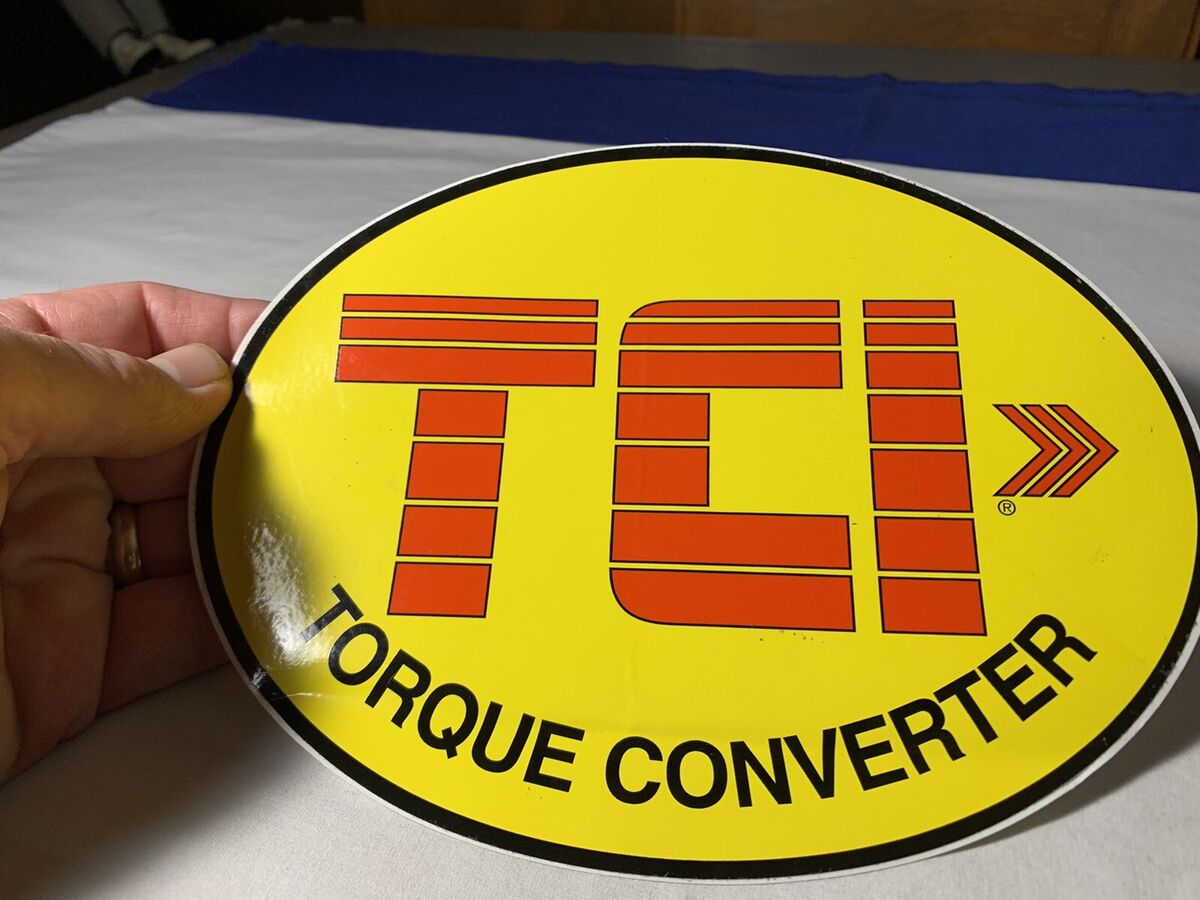This is a detailed color photograph, likely indoors with artificial lighting, showing a posed image of a large, elliptical-shaped sticker prominently displaying the brand "TCI Torque Converter." The sticker has a bright yellow background bordered by a solid black edge. Dominating the center is the brand "TCI" in large, dark orange-red letters, with three rightward-pointing arrows immediately following the "I." Below this, in uppercase black lettering, are the words "Torque Converter."

A Caucasian man's left hand is visible, emerging from the left side of the frame. His thumb is positioned on top of the sticker, while his fingers are behind it, gripping its edge. Notably, he is wearing a wedding ring on his ring finger, and his left thumb's fingernail appears slightly dirty. The background of the image is mostly black with little discernible detail, suggesting it was intentionally kept out of focus to highlight the sticker and the hand holding it. The sticker rests on what appears to be a white cloth atop a countertop or table. The photograph's composition provides a clear, detailed view of the sticker and the hand, capturing the industrial yet straightforward aesthetic of the scene.